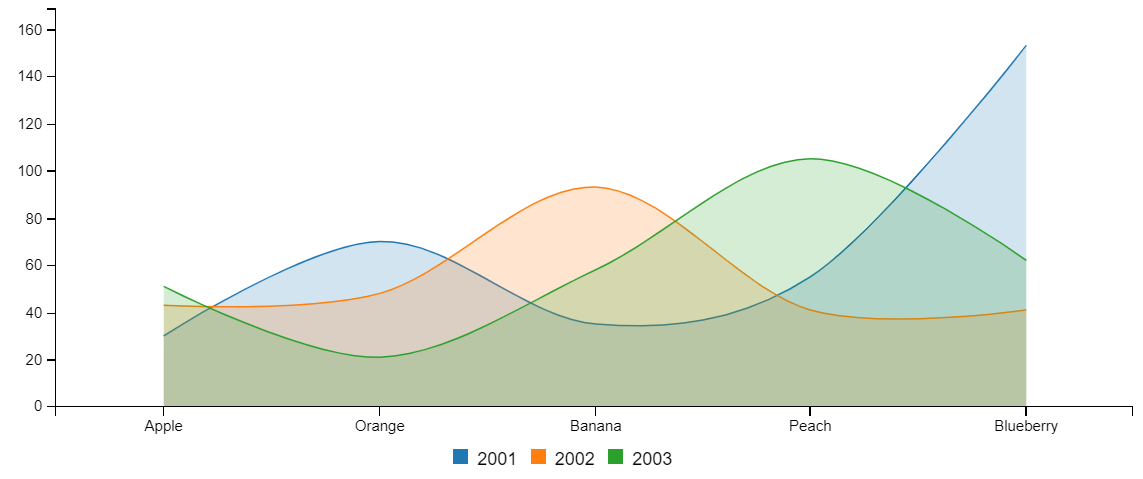This image depicts a detailed bar graph comparing the quantities of various fruits—apple, orange, banana, peach, and blueberry—over the years 2001, 2002, and 2003. Each fruit type is listed along the bottom horizontal axis of the graph in black letters. The vertical axis on the left side of the graph ranges from 0 to 160 in increments of 20. Different colored bars represent different years: blue for 2001, orange for 2002, and green for 2003. These bars illustrate the fluctuating quantities of each fruit across the specified years, with the highest value almost reaching 160, marked by the blue bar for blueberries in 2001. The overall visual data shows a distinct pattern of ups and downs, with a notable spike in blueberry quantities in 2001.